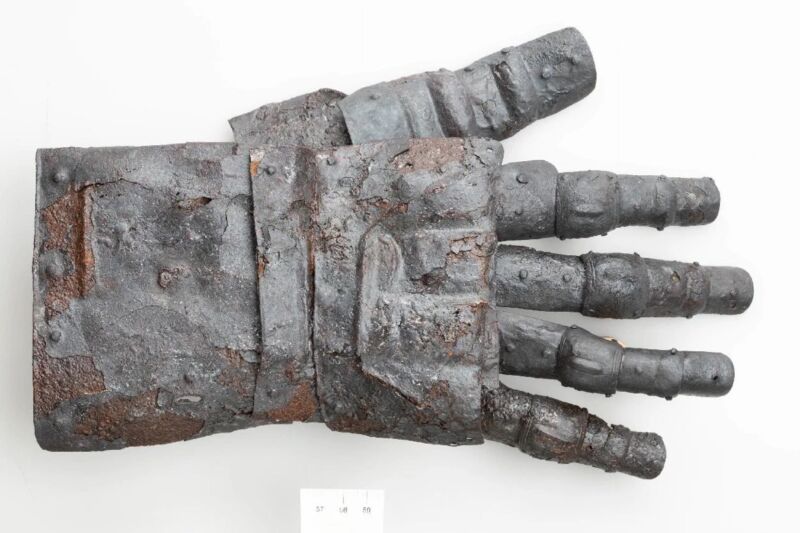The image depicts a right-hand metal gauntlet, likely a museum piece, laid out against a white or light gray background. The gauntlet appears ancient and is primarily a darker shade of silver, interspersed with patches of brown rust, suggesting age and weathering. The gauntlet resembles stone due to its texture but is confirmed to be metal, as evidenced by the visible rust. The fingers of the gauntlet are squared and feature multiple joints and dot-like bumps, and the segmented design includes various layers and riveted sections, giving it an intricate, almost mechanical appearance. Positioned towards the right, the fingers extend from a wrist area on the left. At the base of the gauntlet, there's a small white square of paper with numbers and lines, possibly a museum label, though the text is indecipherable from the photograph. Overall, the gauntlet measures approximately a foot in length and exudes a robust, ancient quality suggestive of medieval armor.